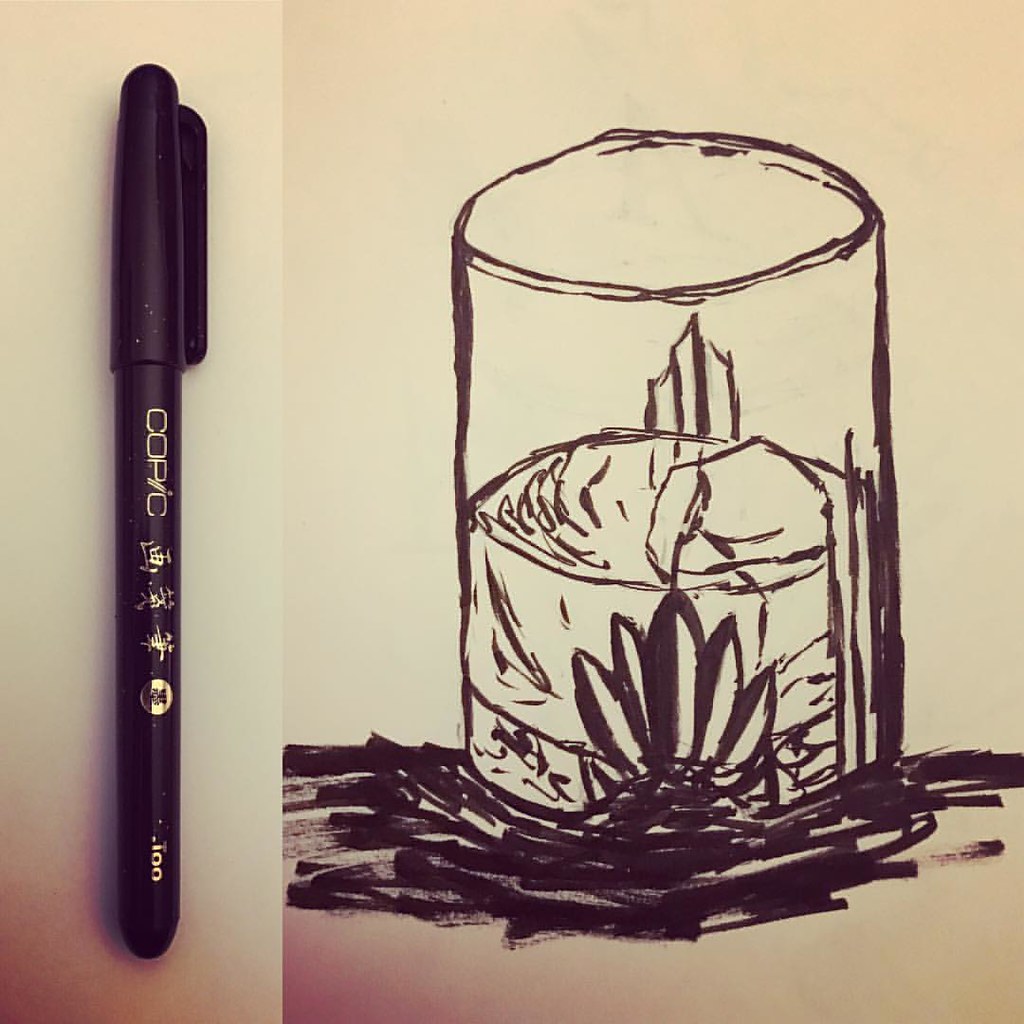On the left-hand side of the image, there is a large black pen with a black cap. In the middle section, silver lettering spells out "Copic," accompanied by some Eastern characters and a silver circle. The bottom part of the pen features some additional text. On the right-hand side of the image, a glass containing a liquid can be seen. At the very bottom of the glass, scattered black particles are visible. The center of the glass showcases what appears to be a flower or multiple leaves fanned out. Additionally, there is a finger or claw-like object, curving from the bottom of the glass to the top.